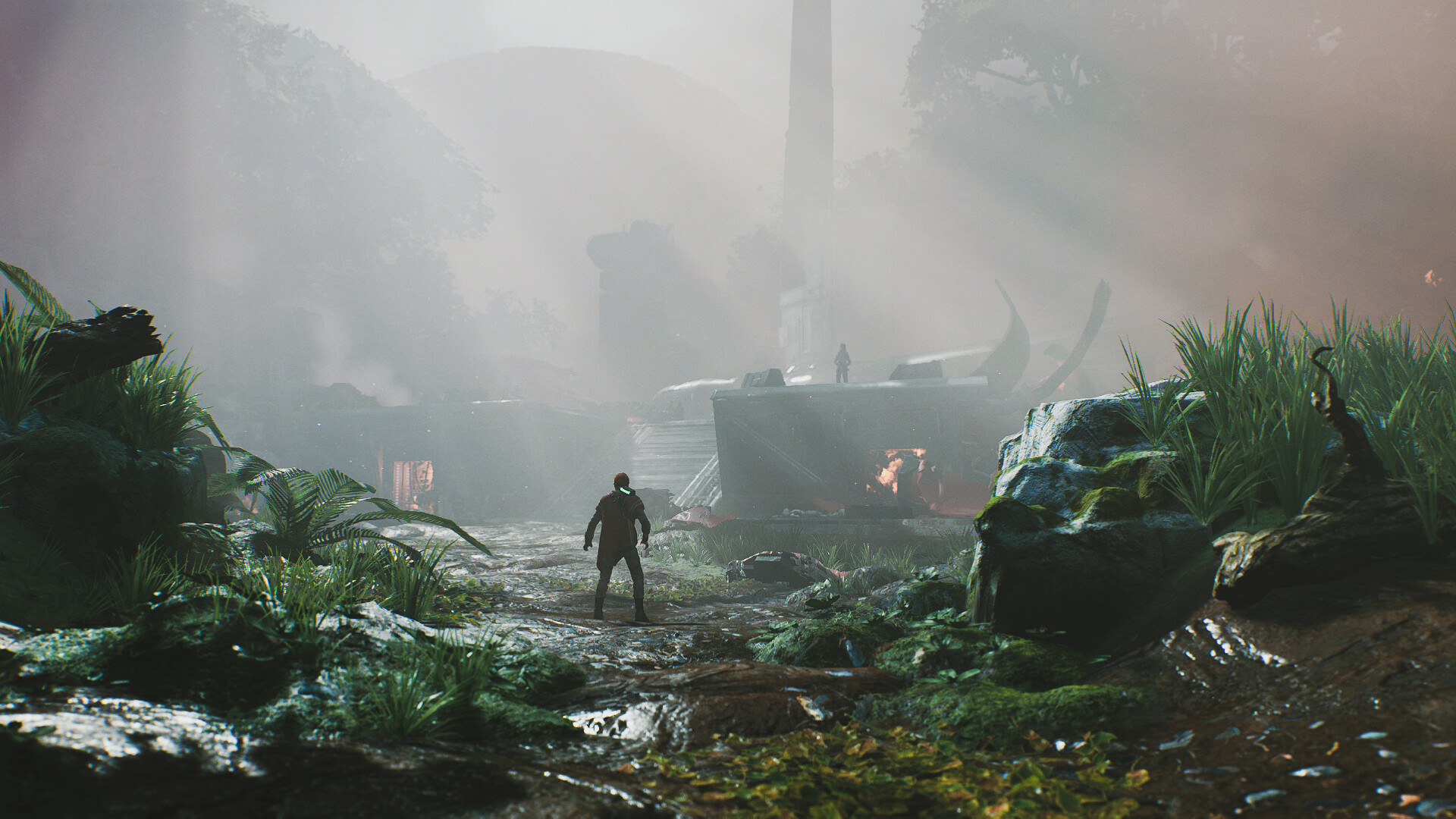This rectangular artwork depicts an intricate outdoor scene. At the center of the composition, the viewer is presented with the back of a person who stands surrounded by lush, green plants. The wet surface beneath the central figure adds to the realism and hints at recent rain or mist. Elevated behind this central figure, another person is visible on a higher platform, contributing to the layered depth of the scene. The background is populated with trees, seen on both the top right and top left of the image, enhancing the natural ambiance. In the distance to the left of the central person, a bright, shining object catches the eye, adding an element of intrigue and wonder to the artwork.